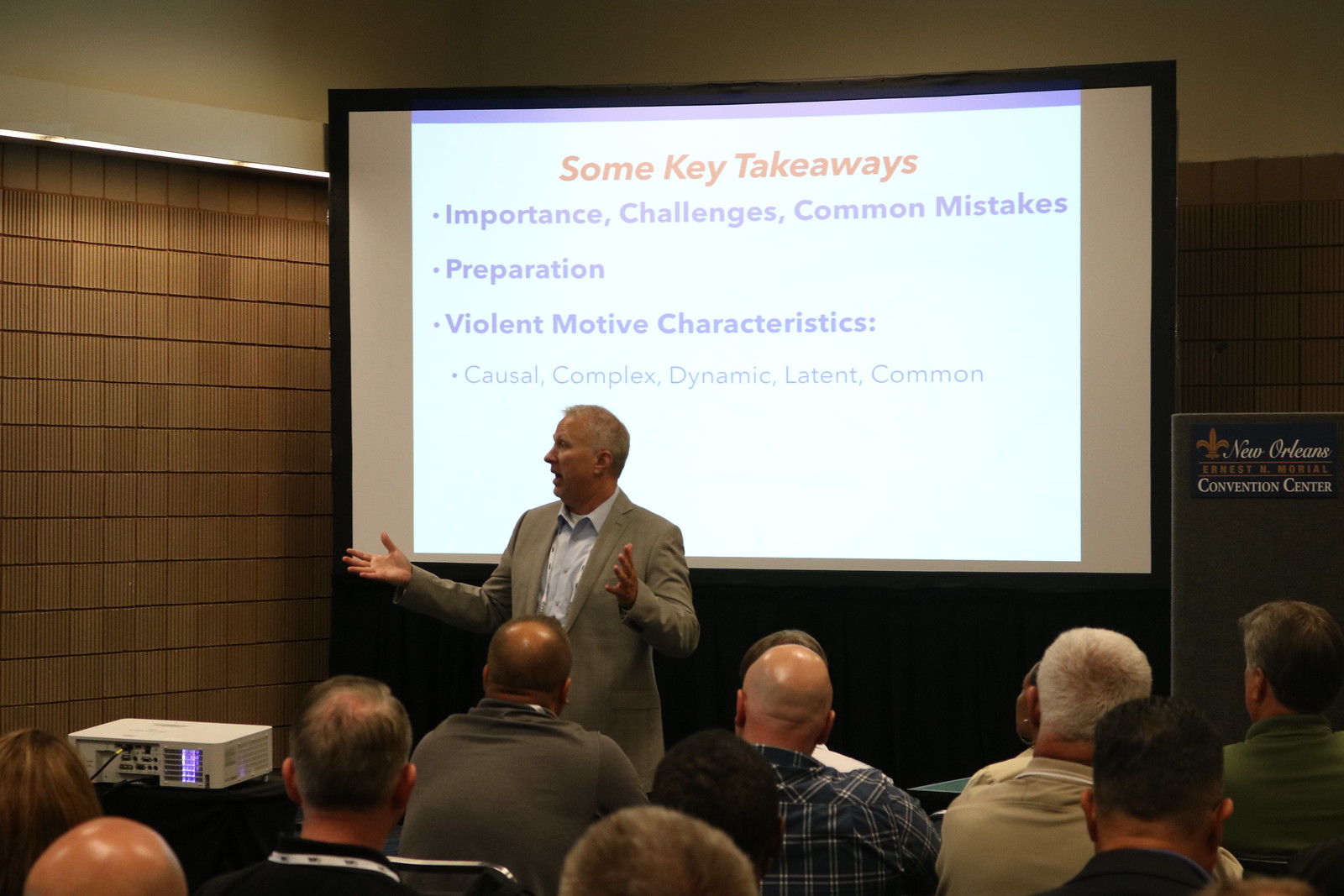In this image, a man with fair skin and hair is giving a presentation at the New Orleans Ernest N. Muriel Convention Center. He is wearing a light gray or tan suit paired with a light blue button-down shirt, and he is gesticulating with his hands while looking to the left. Behind him, a large projection screen displays a PowerPoint slide with a white background. The slide highlights "Some Key Takeaways" in red font and lists several points in blue font, including "importance," "challenges," "common mistakes," "preparation," and "violent motive characteristics," followed by terms like "casual," "complex," "dynamic," "latent," and "common." Seated in front of him are mostly men dressed casually, attentively listening to the presentation. To the right of the image, there is a black barrier or piece of equipment. The setting and attire suggest a formal lecture or workshop, potentially aimed at professionals such as a police group. Additionally, a fleur-de-lis pattern is visible near the text that identifies the location as New Orleans.